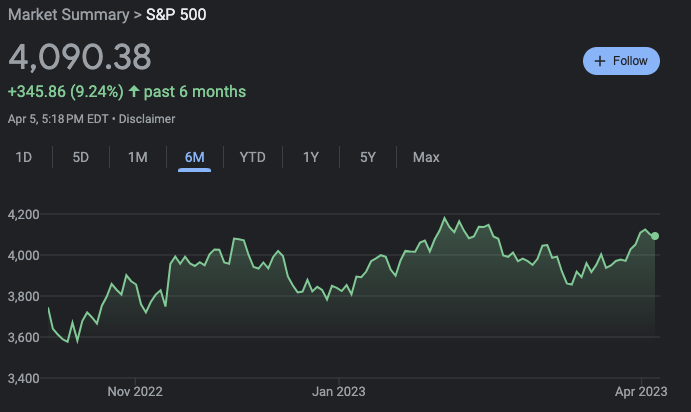This image is a market summary graph of the S&P 500, spanning from November 2022 to April 2023. Set against a sleek black background, the chart depicts the S&P 500's performance trajectory over this period. The graph showcases a general rising trend, despite some periodic declines, indicating an overall upward movement. The data reveals a notable climb from approximately 3,600 points in November 2022 to between 4,000 and 4,200 points by April 2023. The latest data point highlights a value of 4,090.38, reflecting an increase of 345.86 points or 9.24%, signified by an upward arrow. Additionally, the interface allows users to view the market performance over various time frames, including options for one day, five days, one month, six months, year to date, one year, five years, and maximum duration. This detailed visualization aids in comprehending the S&P 500’s performance and trends over the recent months.